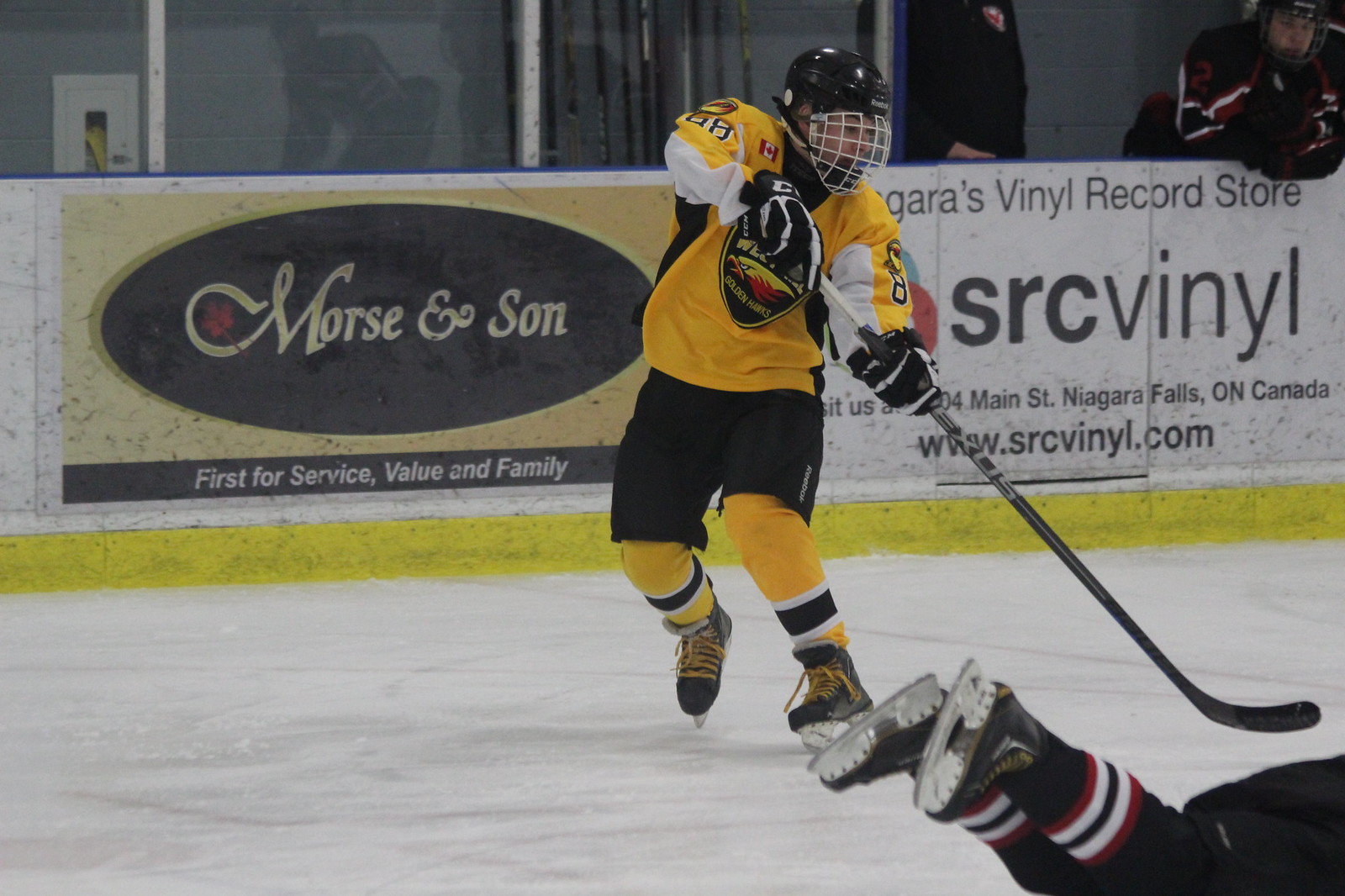In this vivid image taken at an indoor ice hockey game, a dynamic scene unfolds on the icy rink. Central to the composition is a hockey player clad in a striking yellow uniform featuring an eagle emblem, complete with black shorts, yellow and blue socks, and black ice skates with yellow laces. His helmeted head and active stance with a swinging hockey stick suggest a moment of intense action. Nearby, another player lies fallen on the ice, partially out of frame in the bottom right corner. This player wears a predominantly black uniform accented with red and white stripes on his socks. The background is lined with advertisements for "Morse & Son: First for Service, Value, and Family" and "SRC Vinyl: Niagara's Vinyl Record Store," hinting at the game's location in Niagara Falls, Ontario, Canada. Additional players and intricate details in hues of white, black, red, tan, blue, and maroon further enrich the lively atmosphere of this ice hockey rink.